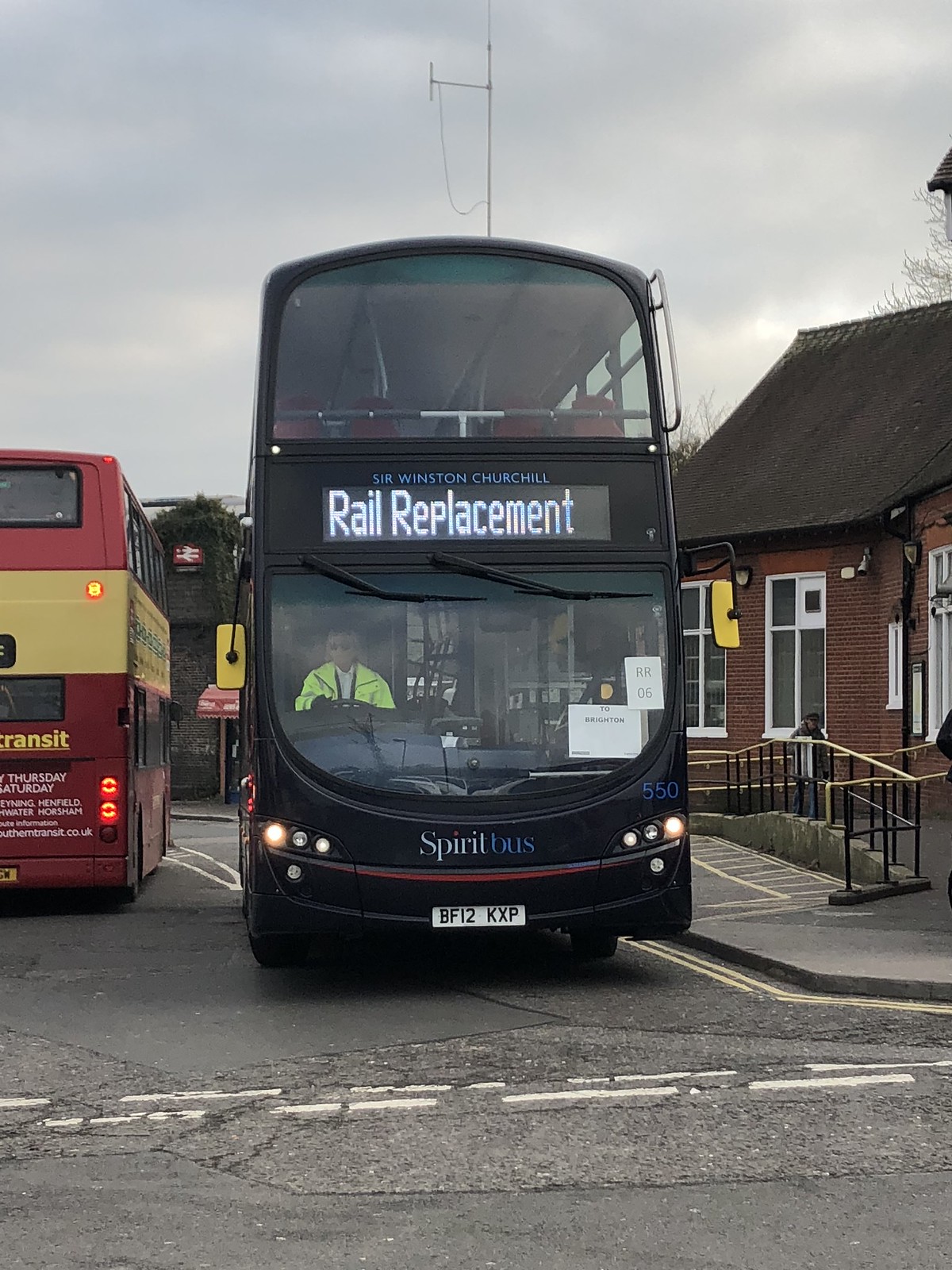The image depicts two double-decker buses at a small bus station in England, identifiable by the license plate and street orientation. The focal bus is black with a clearly visible digital marquee reading "Rail Replacement" and "Sir Winston Churchill." It sports the identifier "Spirit Bus 550" and the license plate BF12KXP. Positioned at the front angle, the viewer can see into the windshield where the bus driver, donned in a bright yellow or lime green jacket, sits at the wheel. This bus appears empty, suggesting it may be out of service or docked for maintenance. Adjacent to this bus is a red and yellow double-decker bus, partially out of frame. The backdrop includes an overcast sky and a red brick building with a black roof, featuring a sidewalk, stairs, and a ramp leading up to a door. The station itself appears quiet, with no passengers in sight, adding to the sense that these buses are temporarily not in operation.